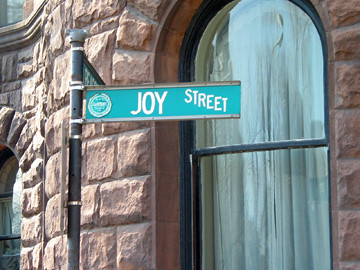The image, which is wider than it is tall, portrays a charming urban street scene centered around a street sign. The sign reads "JOY STREET," with the word "STREET" whimsically angled downward, and both words are styled in bold uppercase letters. The background reveals a coral-colored row house with a distinctive curved facade, reminiscent of a Gaudi-inspired or artsy district. Visible are two windows adorned with white curtains; the first is located on the right side, while the second appears as the facade curves leftward. Both windows are framed uniquely, with square bottoms transitioning into semicircular tops. Completing the scene, an elegant light post stands on the left side of the image, adding to the picturesque setting.